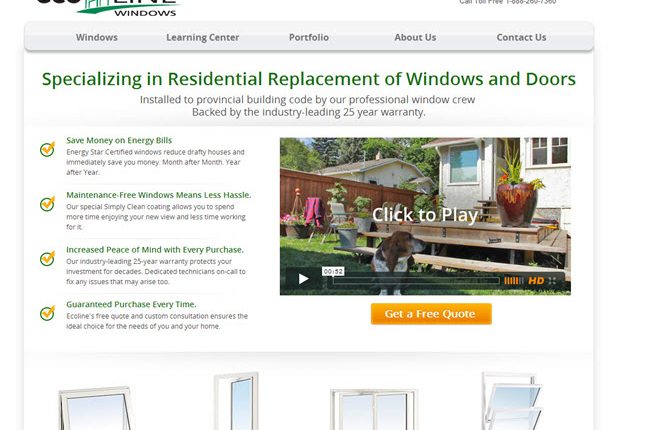This image appears to be a screenshot of a website for a window company. In the upper left corner, there is a company logo next to the word "Windows." Below the logo, there is a navigation bar with options including "Windows," "Learning Center," "Portfolio," and "About Us." Prominently displayed in bold green text is the company's specialization: "Specializing in residential replacement of windows and doors. Installed to provincial building code by our professional window crew. Backed by the industry-leading 25-year warranty."

To the right, there is an inviting image of a house featuring a welcoming porch adorned with a plant. At the center of the porch, there is a brown dog, possibly a basset hound. Overlaid on this image is a "click to play" prompt, suggesting a video about the company can be viewed. Below this image, an orange box labeled "Get a Free Quote" offers a call-to-action for visitors.

On the left side of the main image, and towards the bottom of the page, small thumbnail images showcase various types of windows, further indicating the range of products the company offers.